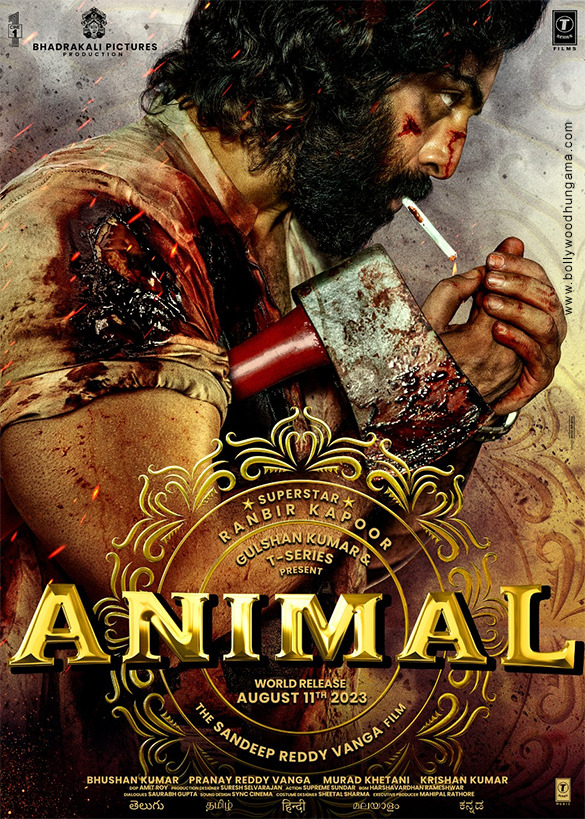This movie poster for "Animal" showcases a dramatic and intense portrait of a rugged man, identified as superstar Ranbir Kapoor. The man has long, curly black hair and a thick black beard, with visible bloodstains on his face, hair, and white t-shirt that's heavily torn and bloodied on the shoulder. His nose and cheek, just below his eye, bear cuts. He appears focused and resilient, lighting a cigarette with his hands, while a bloodied axe is securely tucked under his right armpit. The background transitions from grayish at the top to a bronze hue, adding depth to the image. At the top left, the text reads "Bajiraq Kali Pictures Production," and below the image, a gold print presents "ANIMAL" in large letters. Further text, also in gold, announces "Superstar Ranbir Kapoor, Gulshan Kumar and T-Series Present" alongside "A Sandeep Reddy Vanga Film." The poster indicates a worldwide release on August 11, 2023, in smaller gold print at the bottom. This fierce visual hints at an intense action-packed narrative.